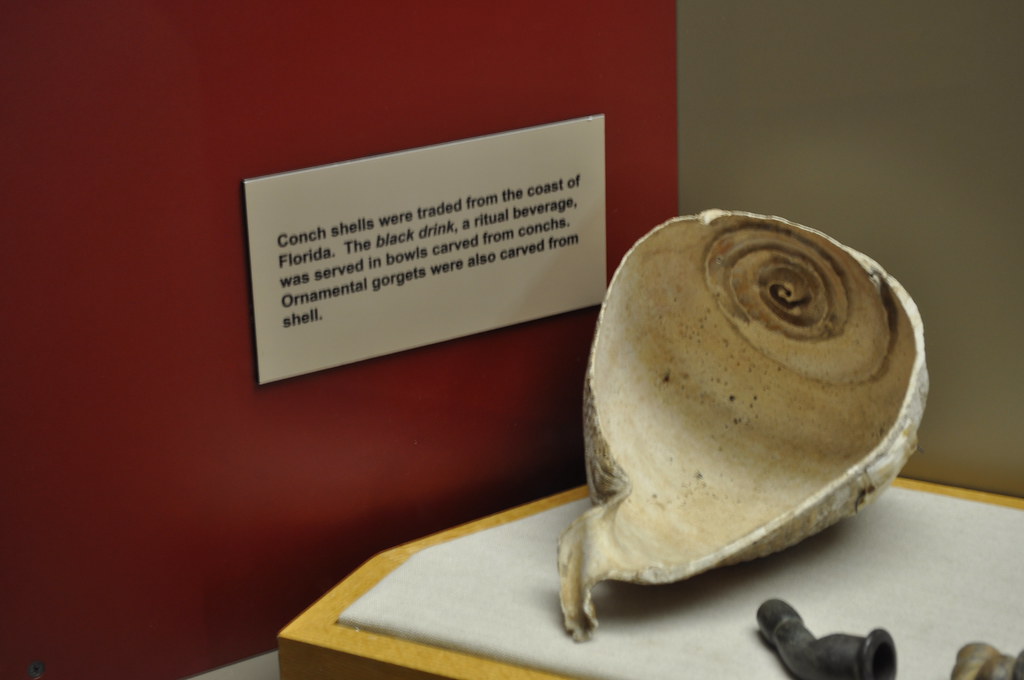The photograph captures a museum exhibit featuring a large, hollowed-out white conch shell, displayed to show its interior, resembling a bowl. The shell rests on a white stand with a yellow outline, situated on a wooden base. The exhibit is set against a backdrop of two walls: one on the left, painted red, with a descriptive caption on a white paper, and the other on the right, in a brown-grey color. The caption reads: "Conch shells were traded from the coast of Florida. The black drink, a ritual beverage, was served in bowls carved from conches. Ornamental gorgets were also carved from shell." Additionally, the bottom right corner of the image shows a tannish-brown and black object. The meticulous setup highlights the cultural and historical significance of the conch shell in the context of Floridian trade and ritual practices.